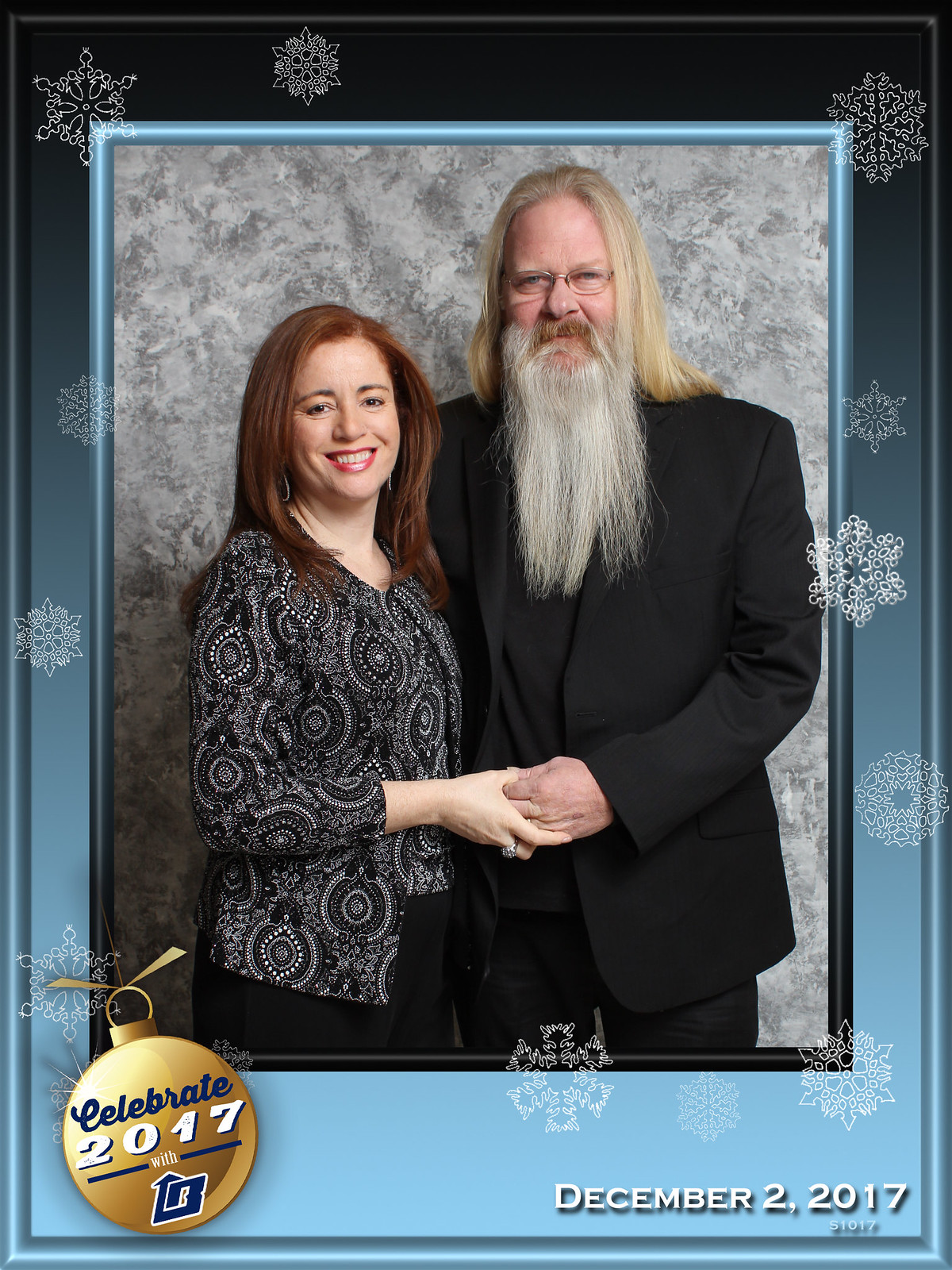The image depicts a joyful couple holding hands, both smiling and facing the camera. The man, much taller than the woman, is on the right. He has long blonde hair, a long beard that reaches halfway down his chest, a goatee, glasses, and wears an all-black suit consisting of a blazer and pants. His beard features gray strands, while his mustache remains brownish. The woman, standing to his left, has long reddish hair cascading to her shoulders. She wears a black top adorned with white circular designs and black pants. The background behind them is white, bordered by a light blue frame decorated with white snowflakes. At the bottom right, white text reads "December 2nd, 2017." Additionally, a gold emblem on the bottom left corner contains the text "Celebrate 2017" along with another emblem beneath it.